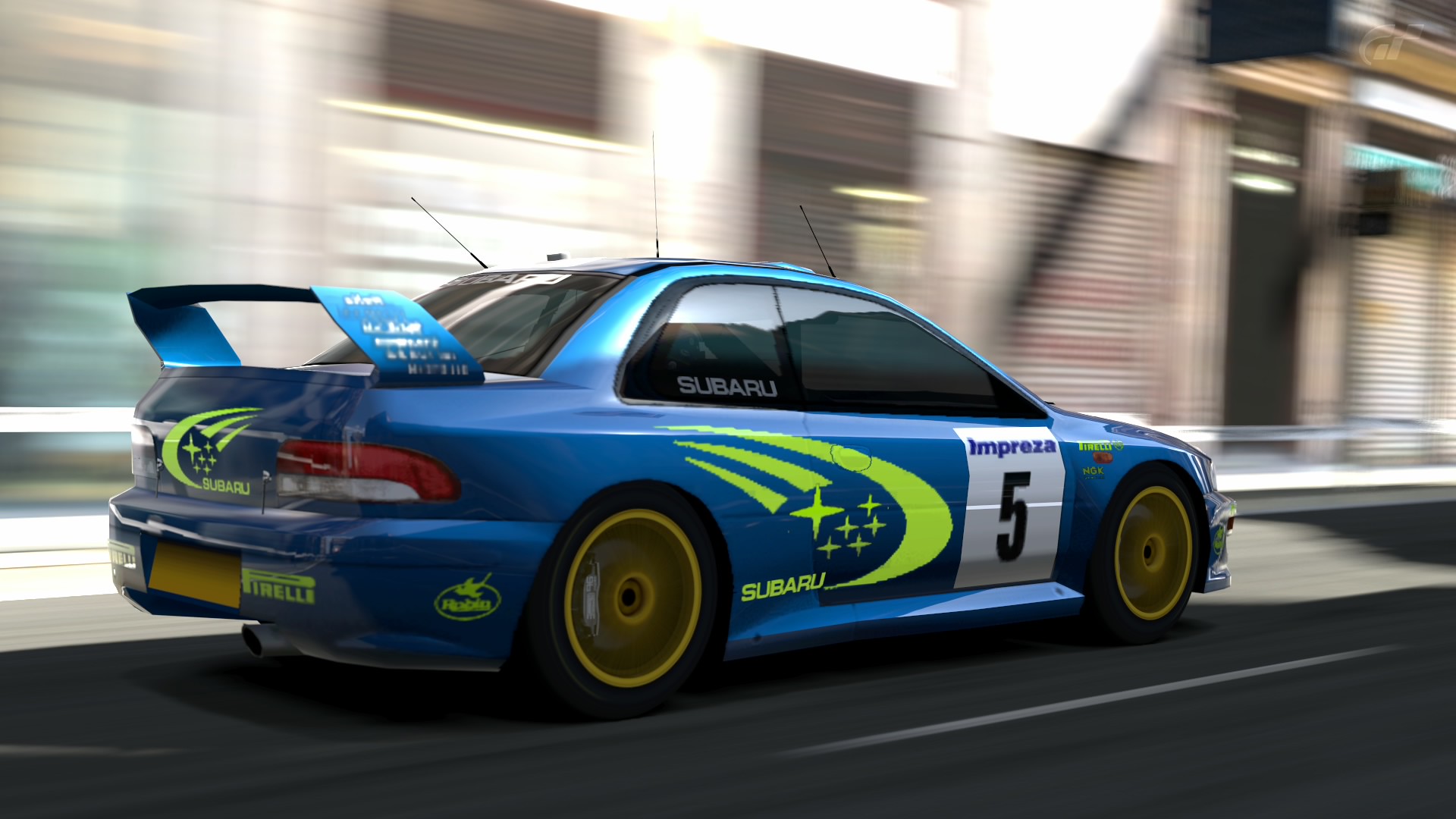This landscape photograph captures a dynamic racing scene featuring a blue Subaru race car on a two-lane road, likely a city track, with a building and garage doors blurred in the background. The car's back end and right side are prominently displayed, with details such as a high, raised blue spoiler and swirled neon green lines accentuating the sleek design. These green lines include outlines of stars and crosses, adding to the striking visual effects on the car. The Subaru logo, boldly written in matching neon green, is accompanied by several advertisement stickers, including one for Ferrari tires. The car sports tinted windows, three antennas on the roof, and yellow rims on black wheels, suggesting it's in motion with the wheels appearing to spin. A white square on the right passenger door frames the words "Impreza" in blue and the number "5" in black. The foreground road has a dashed white line and hints of another lane, emphasizing the speed and movement of the race car.